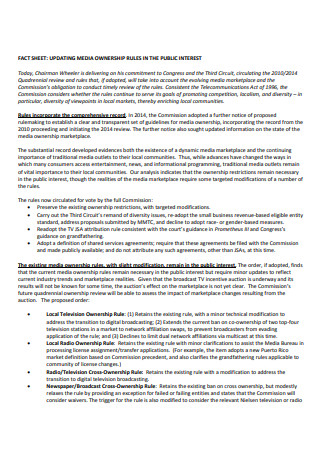This screenshot shows a very blurry and hard-to-read document in portrait mode, featuring an off-white background. In the upper left-hand corner, the text reads "Fact Sheet: Updating Media Ownership Rules in the Public Interest." Further down, the document mentions that today, the chairman is delivering something to Congress and refers to an action by the Third Circuit. The text is very small, gray on white, in italics, making it especially difficult to decipher.

A bolder, underlined section states, "Rules Incorporate the Comprehensive Record." It mentions that in 2014, the Commission adopted a further notice of proposed rulemaking to establish transparent guidelines for media ownership, incorporating records from the 2010 proceeding and initiating the 2014 review. The document sought updated information on the media ownership marketplace and continues with extensive details.

There is another bold section stating, "The Existing Media Ownership Rules with Some Modifications Remain in the Public Interest," followed by bullet points that are also difficult to read due to the small and poorly contrasted text.